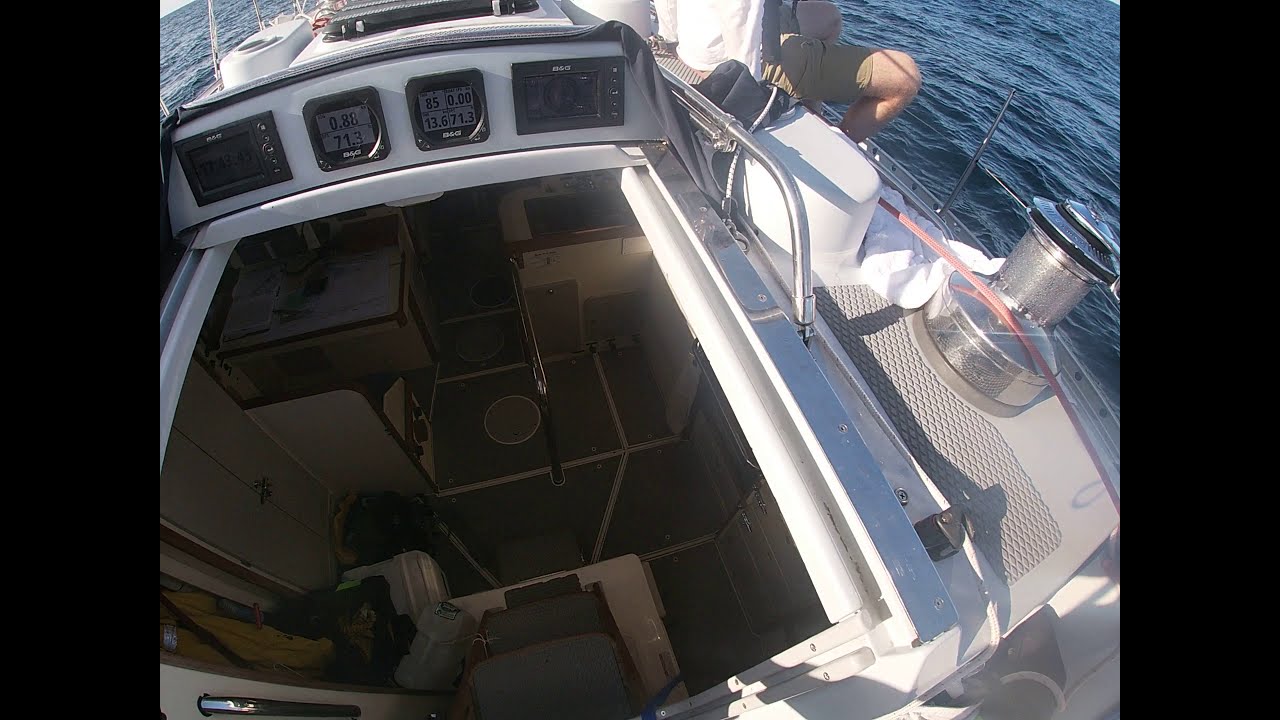This horizontal rectangular image captures a detailed view of a sailboat's interior from above, framed by two thick, black vertical borders which render the colored part as nearly square. The boat's interior is predominantly brown with visible sections including seats and a floor. Dominating the right portion of the image is a white dashboard featuring a gray digital display with black numbers and borders, surrounded by a white surface. Adjacent to this setup, at the boat's edge, sits a partially visible person—probably a man—clad in brown shorts and a white shirt, offering a side view that extends up to their mid-back. This individual appears to be gazing out over the bluish-gray, choppy water visible in the upper right corner. On the right ledge of the boat, a stainless steel canister is placed. Additional elements include a small gray cabinet on the left, and there are hints of gray and brown stairs, plus sectioned-off areas with counters cluttered with papers and various objects. The scene portrays a lived-in, slightly chaotic space, possibly being used for activities like fishing.